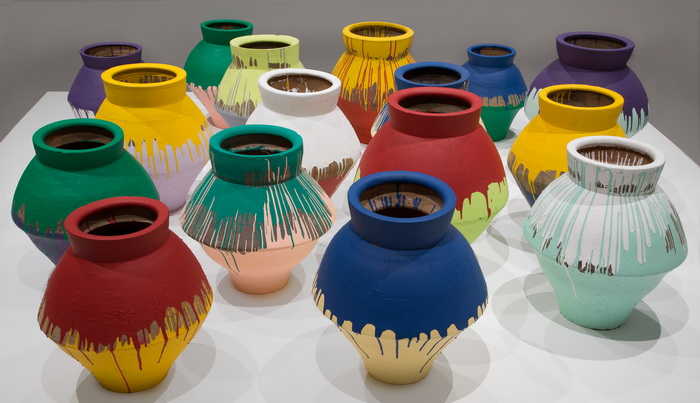The image depicts a collection of 16 ceramic vases arranged on a white table, set against a gray background. Each vase is uniquely painted in an array of vibrant colors, creating a visually engaging display. Notable vases include one with a blue top and yellow bottom, another with a red top and yellow bottom, and several with dripping paint effects. Specific color combinations include mint green and white, red and lime green, green and peach, purple and blue, and various other striking mixture of colors. Among the vases, the one at the back center stands out with its red bottom, yellow top, and red dripping lines creating an intricate design. Overall, the vases feature a variety of colors such as teal, light blue, dark purple, tan, and more, each contributing to the colorful array exhibited on the white table.